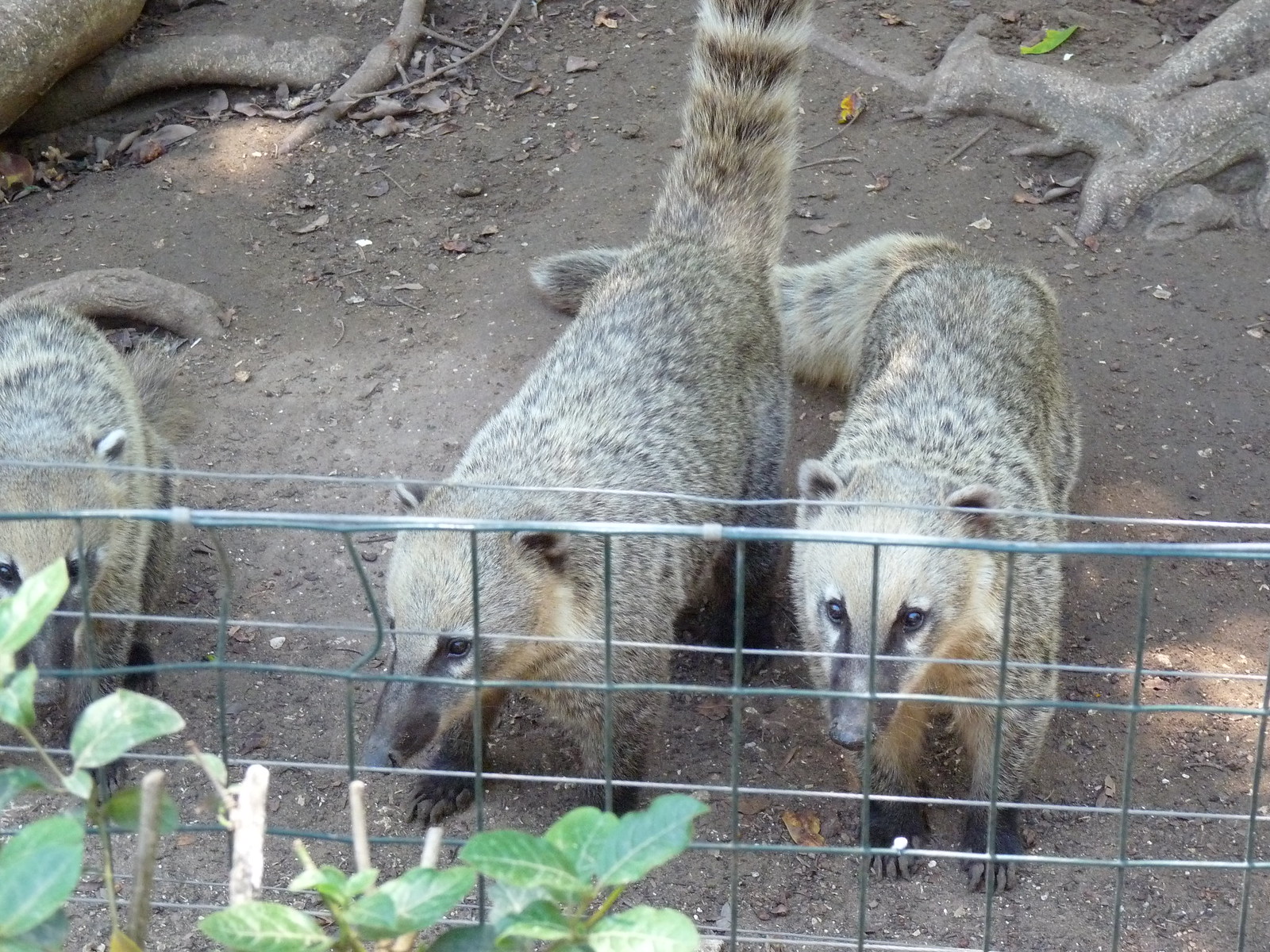In this vertical rectangular image set in a zoo, we observe three dog-raccoon hybrid animals positioned on four legs. They are on gray dirt ground with visible tree roots and scattered gray leaves in the background, suggesting this is their enclosure. One of the animals stands atop a very small, silver-gray fence made of vertical rods intersecting horizontally to form small squares. Each animal has a long snout reminiscent of a dog's, but their short stature and build resemble that of a pug, each probably weighing around 30 pounds and standing one to two feet tall. Their tails, particularly the middle one's which is raised, are furry with distinctive raccoon-like rings of black and gray. The scene is predominantly colored with shades of green, gray, and black, complemented by the natural hues of dirt and tree roots.